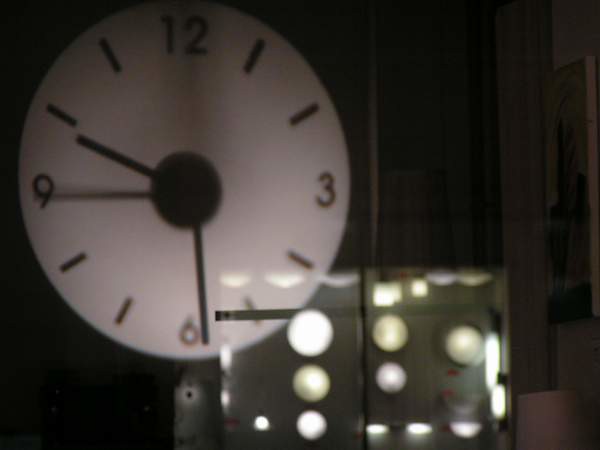This is a close-up, slightly out-of-focus photograph of a circular clock with a white face, housed behind a glass casing. The clock displays black numbers at the 12, 3, 6, and 9 positions, with simple black lines indicating the other hour marks. The clock has black hour, minute, and sweep second hands, with the latter currently crossing over the 9, suggesting a time of approximately 10:29. The clock's face is surrounded by a black frame, which sits on a circular base. The glass casing shows a reflection of cream-colored and white circular lights and buttons, which obscure parts of the clock and create a complex visual effect. To the right, a partial view of a doorway and a painting can be seen, though the details are obscured by reflections and poor lighting. The rest of the background is largely blurred and dark, adding to the overall enigmatic appearance of the photo.